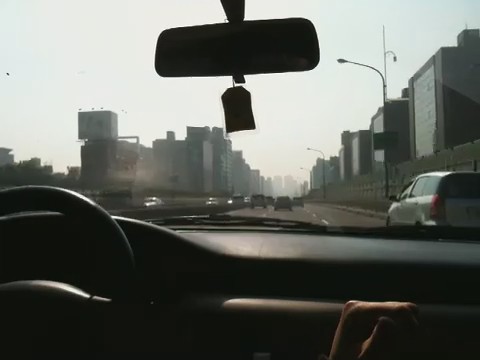In this evocative black and white photograph, we are offered a view from the driver's perspective inside a car. The black steering wheel commands attention at the forefront, complemented by an equally dark dashboard. Suspended from the rearview mirror is a small tag, adding a touch of personalization to the scene. The faint outline of an object is visible on the back seat, its identity obscured but hinting at a story untold. Outside the vehicle, the road stretches ahead, bustling with dynamic energy. Adjacent to the car, a white station wagon cruises along, blending with the urban landscape marked by a large protective fence and several towering brick buildings. The scene is illuminated by street lights that punctuate the light-colored sky. To the left, a cluster of trees bravely stands against the backdrop of more imposing structures. The roads are animated with traffic flowing in both directions, capturing the perpetual motion of city life.